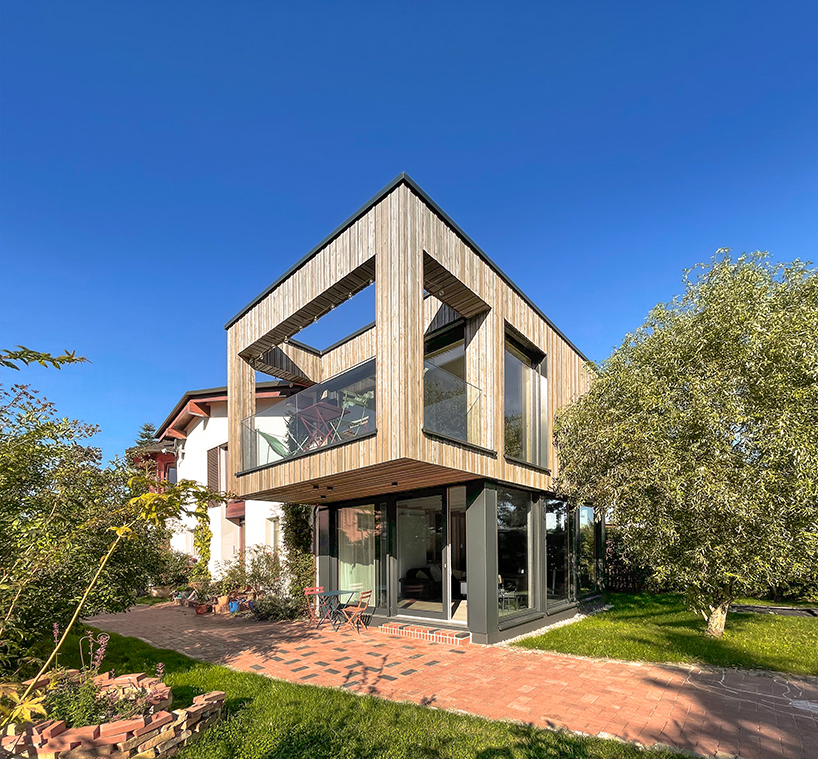The image features a modern, two-story house set against a backdrop of clear blue skies and bright daylight. The house has an intriguing design with many 90-degree angles and extensive use of glass and wood in its construction. The lower level of the house showcases large, floor-to-ceiling glass windows framed in black or gray, providing an open and airy feel. Supporting this level are gray columns that uphold the second story, which slightly protrudes over a brick patio below. 

To the right of the house stands a tree and a patch of grass, while the left features more greenery including shrubs and a brick pot filled with flowers. The walkway leading up to the house starts with red bricks and transitions to grayish-black bricks as it nears the home. The second-story, clad in wood paneling, includes a balcony with glass walls for safety and features a chair. This balcony is notable for its large rectangular openings, providing an unobstructed view of the surroundings. The overall facade of the house combines modern architectural elements with a unique blend of materials and design elements, making it stand out in its picturesque setting.